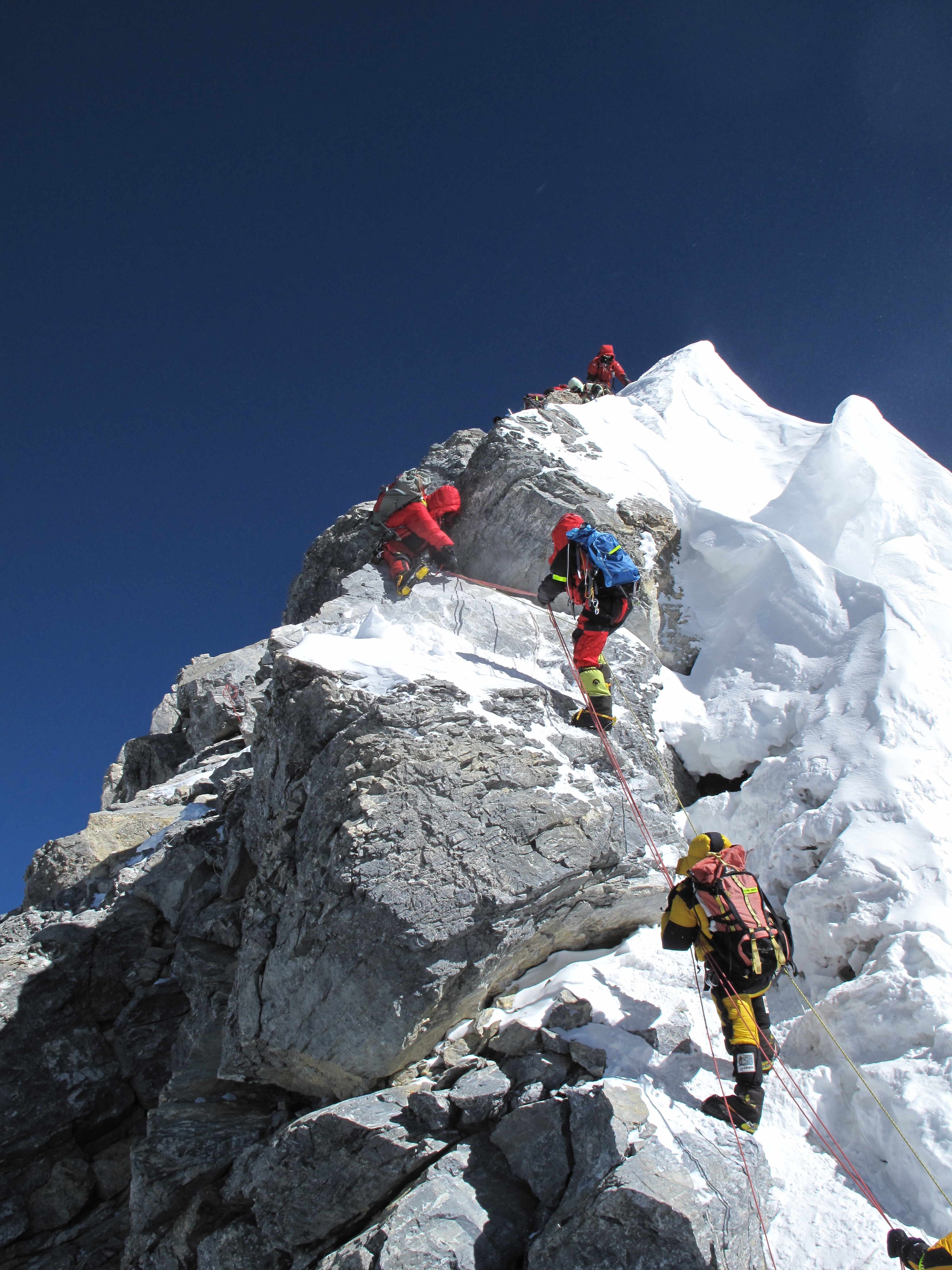The image depicts a daytime color photograph of four climbers ascending a snow-covered mountain, which could be Mount Everest. Set against a clear, cloudless blue sky, the scene shows the climbers connected by a rope, making their way up the steep, treacherous terrain marked by rocks on the left and snow on the right. The climbers are spaced out along the climb, with one already near the summit. Three of the climbers are dressed in red, while the one at the bottom is wearing yellow. The climber at the top has just about reached the peak, while the other three are spread along the rocky ledges below, showcasing their determined progress in this challenging ascent.